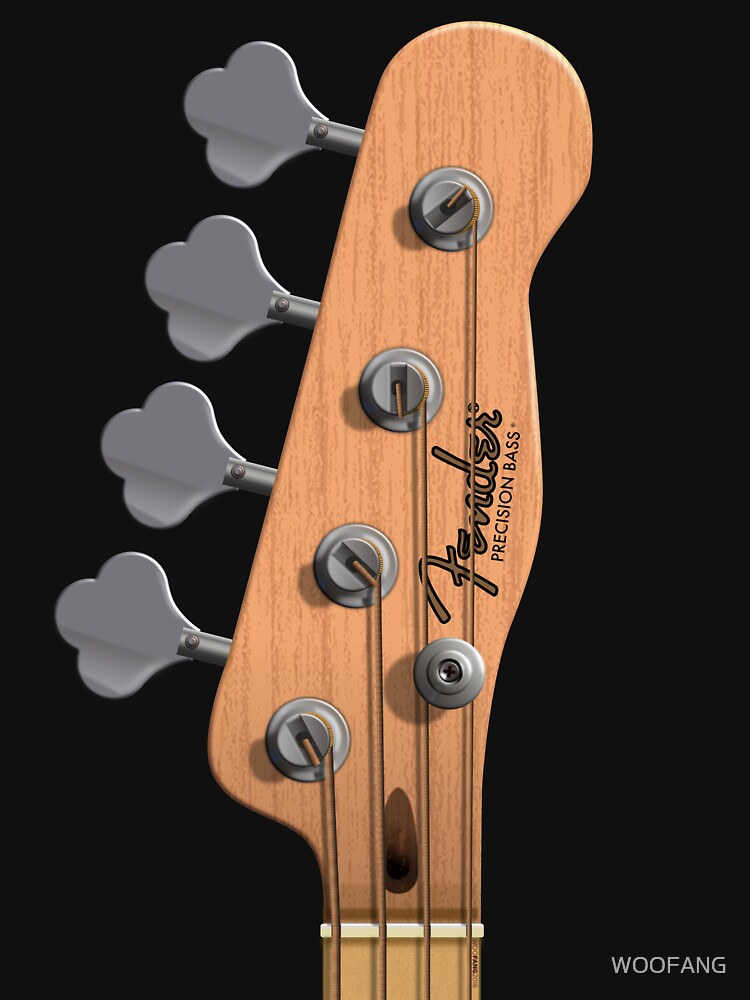This image is an up-close, highly detailed visual of the upper part of a wooden bass guitar, specifically an acoustic Fender Precision Bass. The background is pure black, creating contrast against the guitar’s wooden grain finish. Prominently featured at the top of the neck, where the strings are adjusted, are four grey, clover-shaped tuning knobs. Each knob is attached to a string, with a total of four strings descending down the neck. The tuning knobs, also known as screws, hold the strings in place and adjust their tension. In elegant gold cursive, the brand name "Fender" is inscribed, and beneath it, "Precision Bass" is printed in black capital letters. There's also an angular hole situated among the strings, providing a glimpse of the guitar's intricate structure. On the bottom right-hand corner of the image, the watermark "Wu Fang" is written in white. The neck of the guitar features horizontal bars, though only one white fret is visible in this close-up. Near the third and fourth strings, a small silver bolt adds a final touch of detail to this meticulous depiction of the guitar’s headstock.